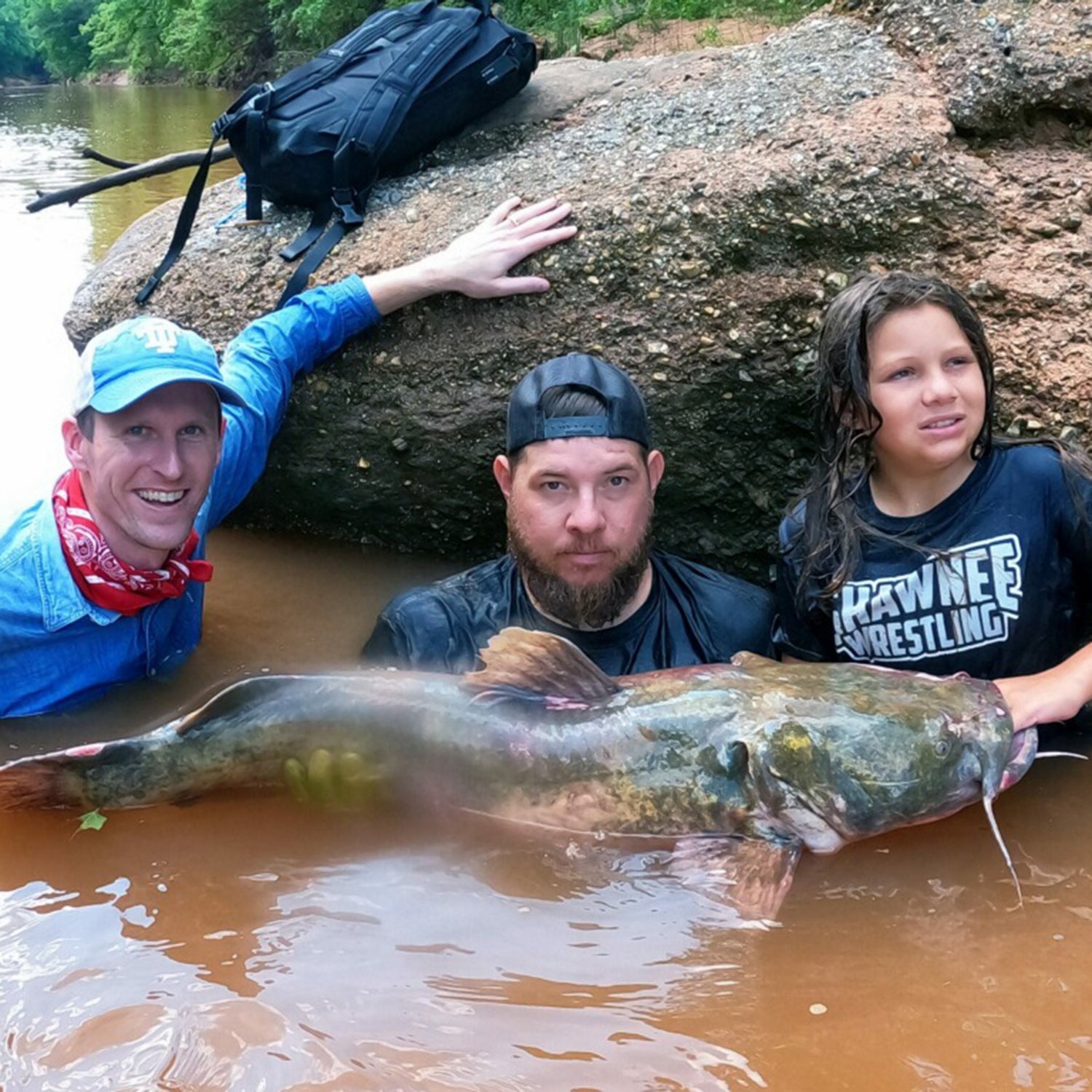In this captivating outdoor scene set against a backdrop of a tree-lined embankment, three individuals are submerged up to their shoulders in murky river water, leaning against a large brown boulder. They proudly display a massive catfish, stretching across all three of them as if it were a prized trophy. On the left, a smiling man in a blue denim shirt, adorned with a red neckerchief, and wearing a blue cap, has his left hand resting on the rock. His enthusiasm is palpable. In the middle, a stern-faced man with a beard and mustache looks directly at the camera, sporting a soaked dark blue shirt and a backward black baseball cap. To the right, a young girl with long black hair and a Shawnee wrestling shirt seems to be looking away, intriguingly placing her hand in the fish's mouth. Atop the boulder, a backpack and a tree branch complete the composition, framing this adventurous and triumphant capture moment.